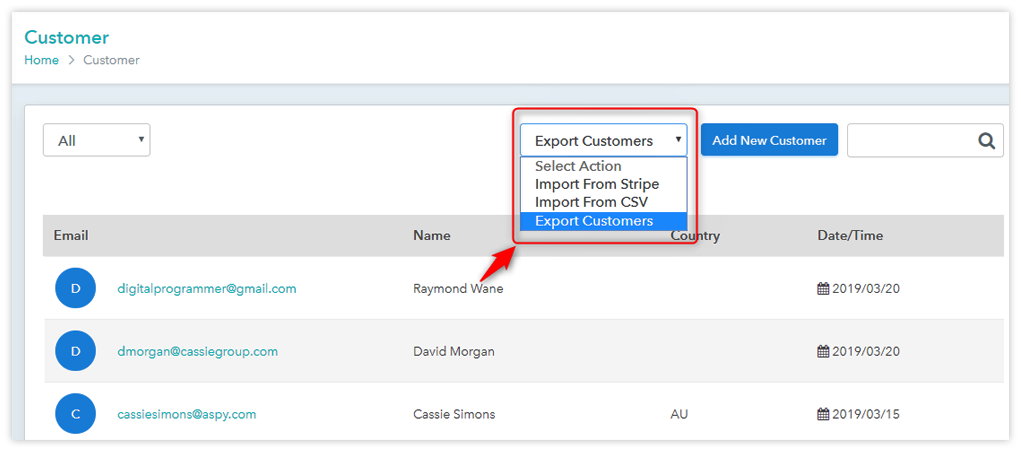This detailed caption provides a comprehensive description of a user interface on a customer management platform or page:

---

The image displays a screenshot of a customer management platform. At the very top, a white rectangular border stretches from left to right. In the left-hand corner of this border, the word "Customer" is displayed in turquoise blue, followed by the word "Home", and a right-facing caret (greater than sign). The caret and the word "Customer" are in gray, while "Home" is in turquoise.

Below this, there is a gray background box occupying a significant portion of the page. Inside this gray box, there is a prominent white rectangular box. In the top left corner of this white box, a drop-down menu labeled "All" in black text is present. On the far right side, another drop-down menu reads "Export Customers". This menu is expanded, revealing options underneath: "Select Action", "Import from Stripe", "Import from CSV", and "Export Customers". The "Export Customers" option is highlighted in blue, while the entire drop-down menu and options are enclosed in a red outline.

To the right of the drop-down menu, there is a blue rectangular button with the text "Add New Customer" in white. Adjacent to this button, on its right, is an empty search box with a black magnifying glass icon.

Moving down, there is a horizontal gray rectangular border box with column headers. These headers are "Email" in black, followed by "Name", "Country", and "Date/Time". 

Under the "Email" header, three email entries are listed:
1. The first entry features a blue circle with a white letter "D" inside, followed by "DigitalProgrammer@gmail.com" in blue font. Under the "Name" header, it reads "Raymond Wayne" in black font. A red arrow points from "Raymond Wayne" towards the "Export Customers" option in the drop-down menu. The "Country" field is empty, and under the "Date/Time" header, a calendar icon is displayed next to the date "2019/03/20".

2. The second entry also features a blue circle with a white letter "D" inside, followed by "DMorgan@CatholicGroup.com" in blue. Under the "Name" header, it reads "David Morgan" in black font. The "Country" field is empty, and the "Date/Time" shows a calendar icon next to "2019/03/20".

3. The third entry shows a blue circle with a white letter "C" inside, followed by "CassieSimons@ASPY.com" in blue. Under the "Name" header, it reads "Cassie Simons" in black. Under "Country", it states "AU", and under the "Date/Time" section, a calendar icon is next to the date "2019/03/15".

---

This caption effectively provides a clear and detailed description of the user interface elements and their arrangement.